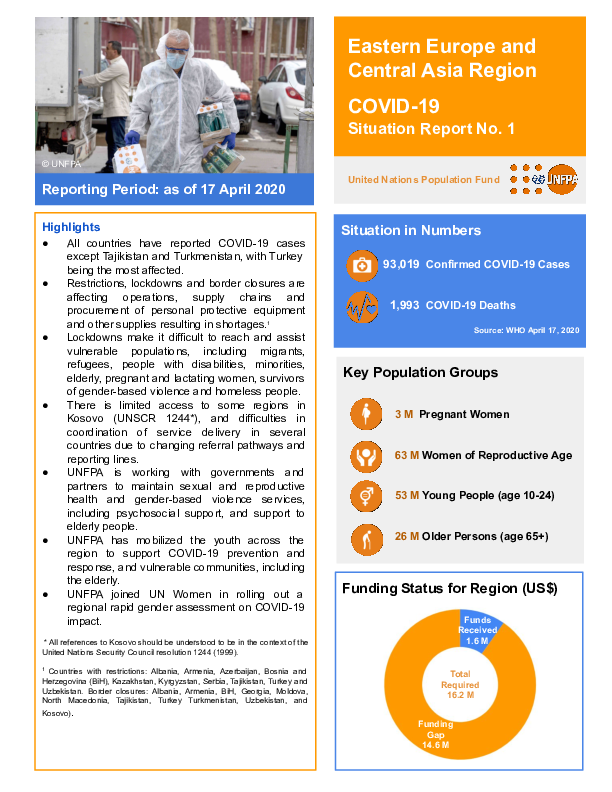A detailed COVID-19 situation report is depicted on the screen.

In the upper left-hand corner, there is a photograph of a doctor wearing a mask and carrying several items. Behind him, a truck is visible, alongside another person standing by the truck. Below the photograph, a blue banner reads "Reporting period as of 17 April 2020."

Beneath this blue banner, there is an orange border containing the word "Highlights" in blue font. This section lists seven bullet points in black font, providing detailed highlights.

To the right of the photograph, there is an orange box with white text that reads "Eastern Europe and Central Asia region, COVID-19 Situation Report Number One." Below this box, a white banner with orange text states "United Nations Population Fund."

Further down, a blue box with white text displays the current "Situation and Numbers": 
- 93,019 confirmed COVID-19 cases
- 1,983 COVID-19 deaths

Next to each statistic, there are orange circles marking the numbers. 

Underneath this statistics box, there is a section titled "Key Population Groups," showcasing four icons representing:
- Pregnant women
- Women of reproductive age
- Young people
- Older persons

In the lower right-hand corner, there is a white square with a blue border. This section, labeled "Funding Status for region (USD)," includes a chart depicting the current funding situation.

This comprehensive report provides a clear snapshot of the COVID-19 impact and response in the Eastern Europe and Central Asia region as of April 17, 2020.